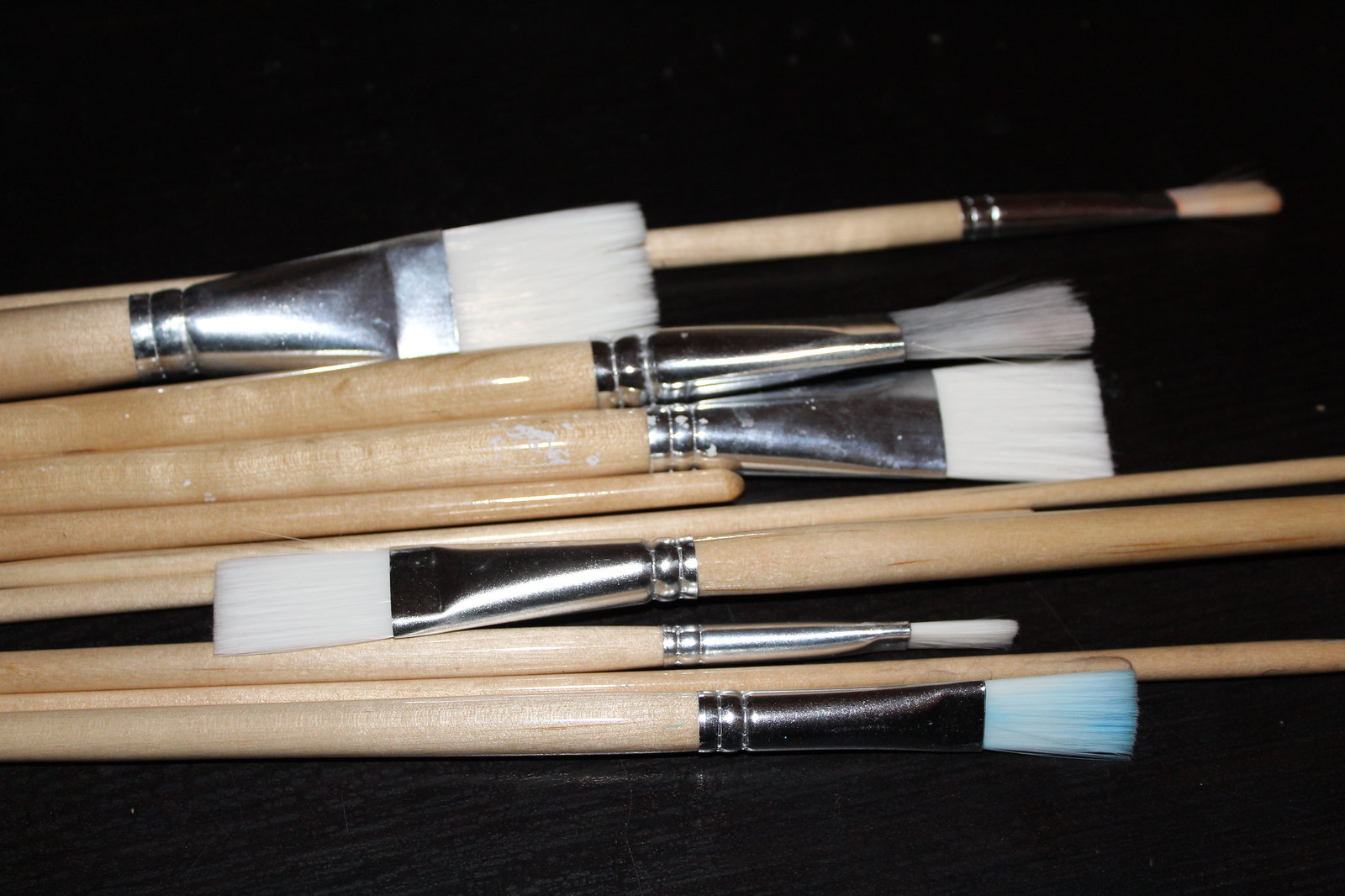This up-close, zoomed-in photograph showcases a collection of high-quality artist paintbrushes laid against a dark background. The brushes feature blonde wood handles, possibly oak, beautifully coated with a shiny varnish. Each brush is adorned with a sleek silver bezel attaching the bristles to the handle. The bristles vary in color, with most being pristine white, though some deviate slightly—including a brush with light gray bristles, another with tan bristles, one with a hint of pink, and another with a touch of light blue. The brushes come in an assortment of sizes and shapes, ranging from small, narrow tips to larger, flat, broad heads, all impeccably clean and new, suggesting they have yet to be used. Some brushes are oriented to the left, while others face to the right, enhancing the dynamic composition of the image.